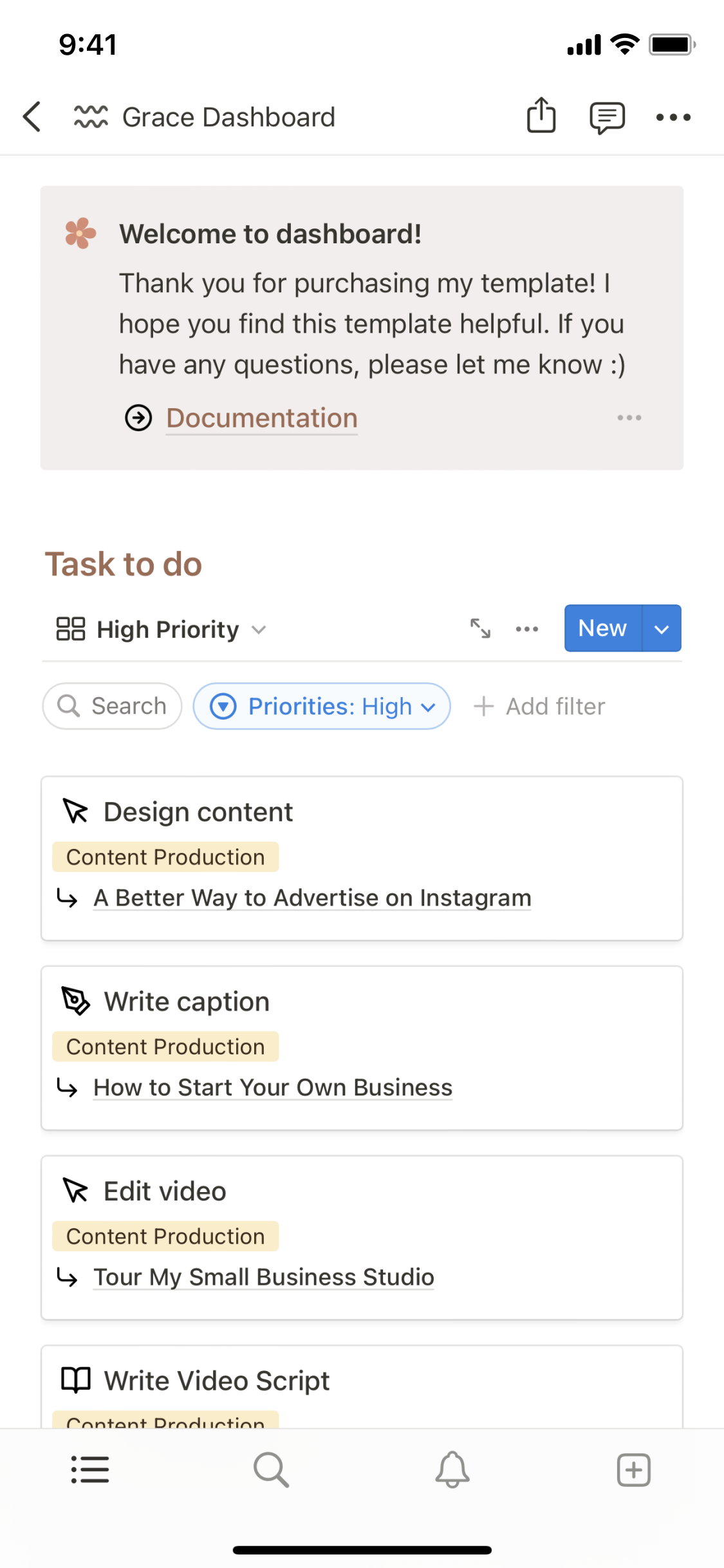The screenshot is taken from a cell phone's display with the time shown as 9:41 in the top-left corner. The top-right corner indicates full cellular reception with four bars, connected Wi-Fi, and a fully charged battery. Below this status bar, there’s a navigation arrow pointing left, two wavy lines, and the header "Grace Dashboard" written in clean, modern typography. This is followed by a set of icons indicating download, reply, and more options (three horizontal dots).

Beneath this header, there’s a gray square with a small pink flower icon at the top. The text within the gray square reads: "Welcome to Dashboard. Thank you for purchasing my template. I hope you find this template helpful. If you have any questions, please let me know." This message is punctuated by a smiley face emoticon.

Below the welcome message, a black circle contains an arrow pointing to the right, adjacent to the text "Documentation."

The next section outlines tasks to be completed, labeled as high priority. This task list includes:
- "New, Search, Priorities High"
- "Add Filter"
- "Design Content"
- "Content Production"
- "A Better Way to Advertise on Instagram"
- "Write Caption"
- "Content Production"
- "How to Start Your Own Business"
- "Edit Video"
- "Content Production"
- "Tour My Small Business Studio"
- "Write Video Script"
- "Content Production"

The image only shows the first part of the task list, with the rest cut off at the bottom.